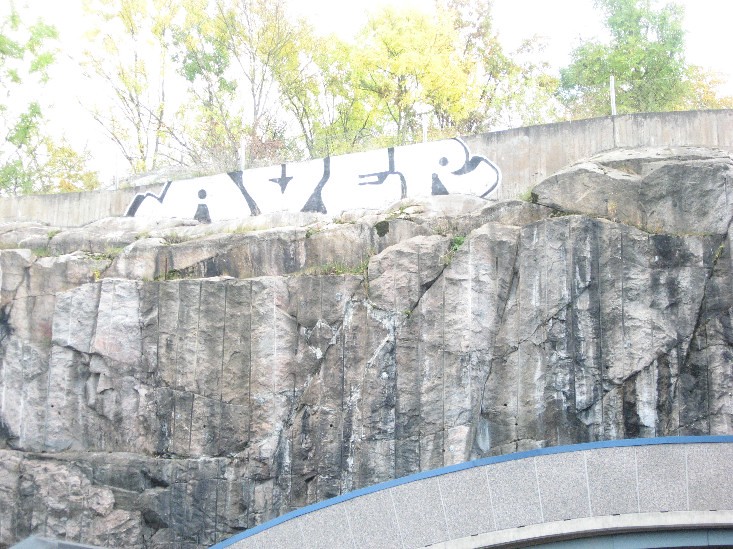The image captures an outdoor scene centered on a stone bridge with rock-faced walls. The bridge, prominently positioned in the middle of the frame, features a concrete section with bold, black and white graffiti near the top center, spelling out "A-V-E-R." The lower right portion of the image showcases part of the bridge's sturdy rock wall. Above the bridge, the overexposed top third of the image reveals a backdrop of sparse green and chartreuse trees, their colors somewhat washed out due to the bright sunlight. Power lines can be faintly seen behind the bridge. The colors in the picture include various shades of green from the trees, along with white, black, gray, and hints of tan and light blue in the surroundings. The photograph appears to have been taken outdoors in the middle of the day, from the perspective of someone standing nearby the bridge.